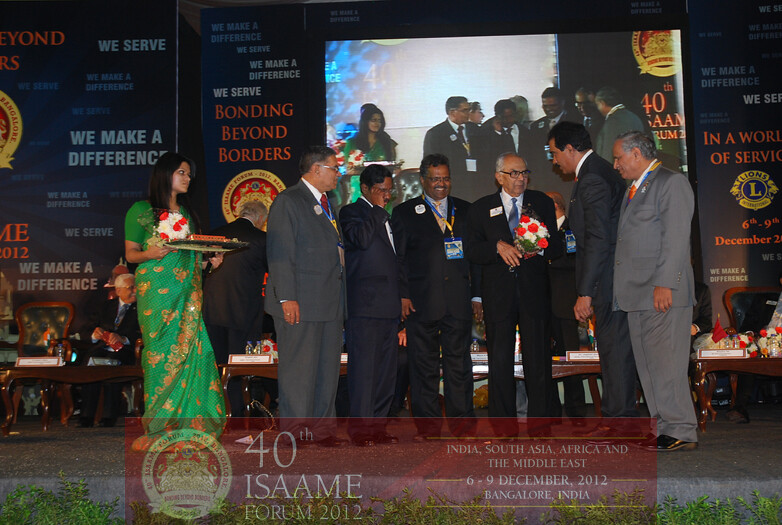This color photograph captures a commemorative event taking place on a gray stage within a convention room, likely in Bangalore, India. Featured prominently in the image are several elements, including a transparent red footer at the bottom containing a seal on the left and detailed event information to the right, reading: "40th ISAAME Forum 2012, India, South Asia, Africa, and the Middle East, 6 to 9 December 2012, Bangalore, India."

On the stage, positioned to the left, stands a woman of Indian descent in a long, dark green sari adorned with gold flowers. She holds a platter with red and white roses. To her right, arranged in a semi-circle, are six men of Indian descent dressed in gray or black business suits. Particularly noticeable is the elderly man in the center-right, who is bald on top with white hair and holds a bouquet of red and white roses, suggesting a moment of recognition. The man next to him has his hand on the elderly man's shoulder, and the rest are attentively facing him.

The stage background is predominantly black with repeating white text that reads, "We make a difference. We serve. Bonding beyond borders." There are dining chairs in the background, indicating the venue's interior setting. Additionally, a large screen above the stage displays an enlarged image of the individuals on the stage, making the details more visible to the audience. A circular Lions Club International logo also features prominently in the background. The overall photographic style is representational realism, emphasizing the details and context of the event.